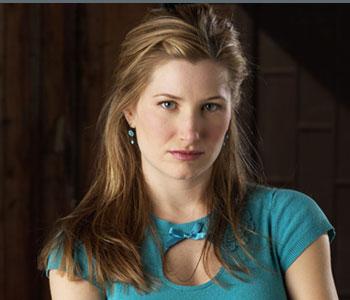The image features a light-skinned woman with long, slightly wavy, dirty blonde hair that falls over her shoulders. She has striking dark blue eyes and turquoise dangling earrings, each with a larger and a smaller glob. Her expression is serious, with her lips set together. She is wearing a turquoise blue short-sleeved dress that ends just over the shoulders. The dress has a distinctive cut-out oval around her upper chest area, revealing the top of her cleavage, and features a bow-tie detail. Her face is adorned with makeup, providing a blush-enhanced look. The background appears to be indoors, with a dark setting that includes a brown wall featuring a brick design, and some shadowing at the top right.